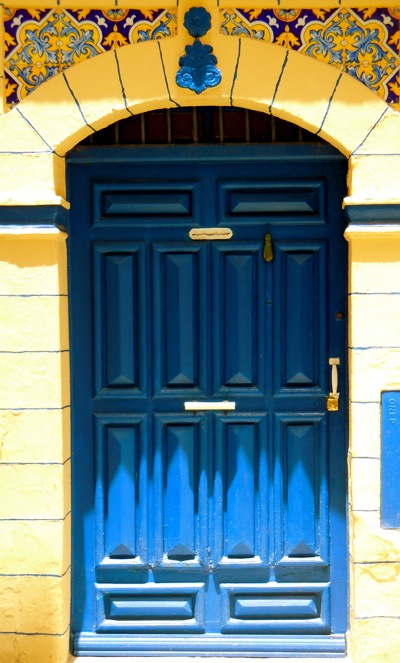This captivating painting features a closed, arched door that takes center stage. The door, painted in shades of blue, transitions from a dark blue hue at the top to a lighter blue at the bottom, suggesting illumination from an unseen light source. A light yellow handle accentuates the door, harmonizing with the light yellow walls that surround it. Above the door, an array of intricate patterns in blue, yellow, orange, white, and touches of green add a vibrant, detailed contrast, enhancing the painting's overall complexity and allure.